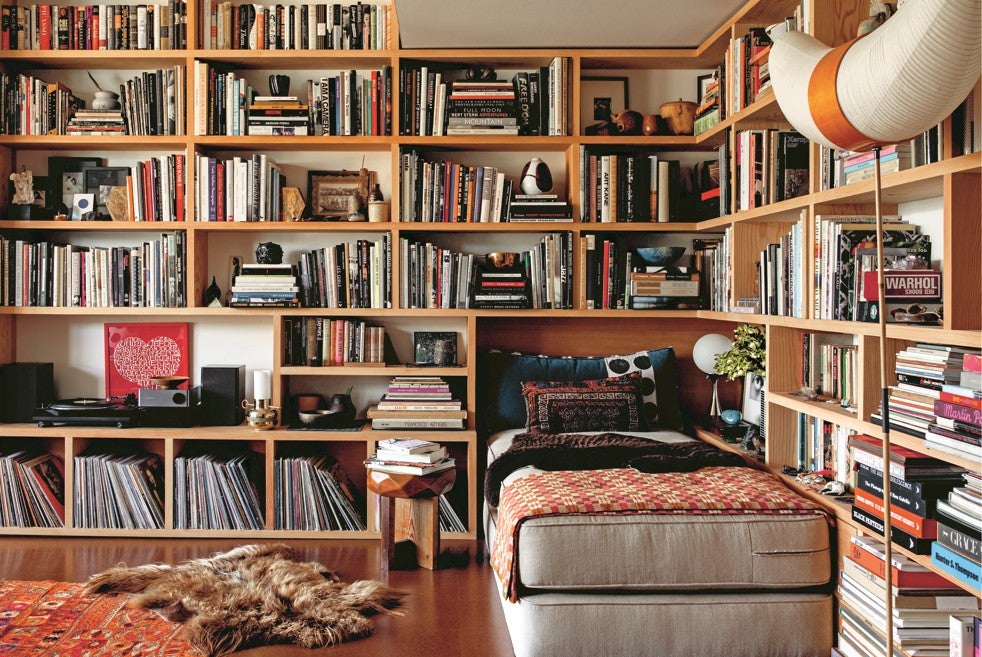This photograph captures a cozy and eclectic room that merges the functionality of a bedroom and a study. Dominating the space are floor-to-ceiling bookshelves made from light to medium brown wood, wrapping around two sides of the room and filled with an extensive collection of books, magazines, and an array of decorative vases, jars, and knickknacks.

In one alcove, two large cushions or mattresses are placed side by side directly on the floor, creating a comfortable sitting or resting area adorned with a variety of pillows and a checkered pink and ivory blanket, with another, darker blanket folded neatly. A small lamp on the adjacent shelf provides a warm glow to this inviting nook.

Below, a dark wooden floor is partially covered by both a red area rug and a luxurious, faux-fur or animal pelt-style rug. A wooden stool next to the mattresses supports stacks of books, underscoring the room’s scholarly atmosphere. A turntable and two speakers are neatly integrated into one of the shelves, accompanied by a picture of a heart and a prominent sign that reads "Warhol," adding a touch of modern art flair.

Scattered throughout the space are little pots, jars, and other personal artifacts, enhancing the room’s warm and lived-in feel. Overall, the room reflects the personality of an avid reader and a lover of both literature and music, combining functionality with a sense of creative expression.